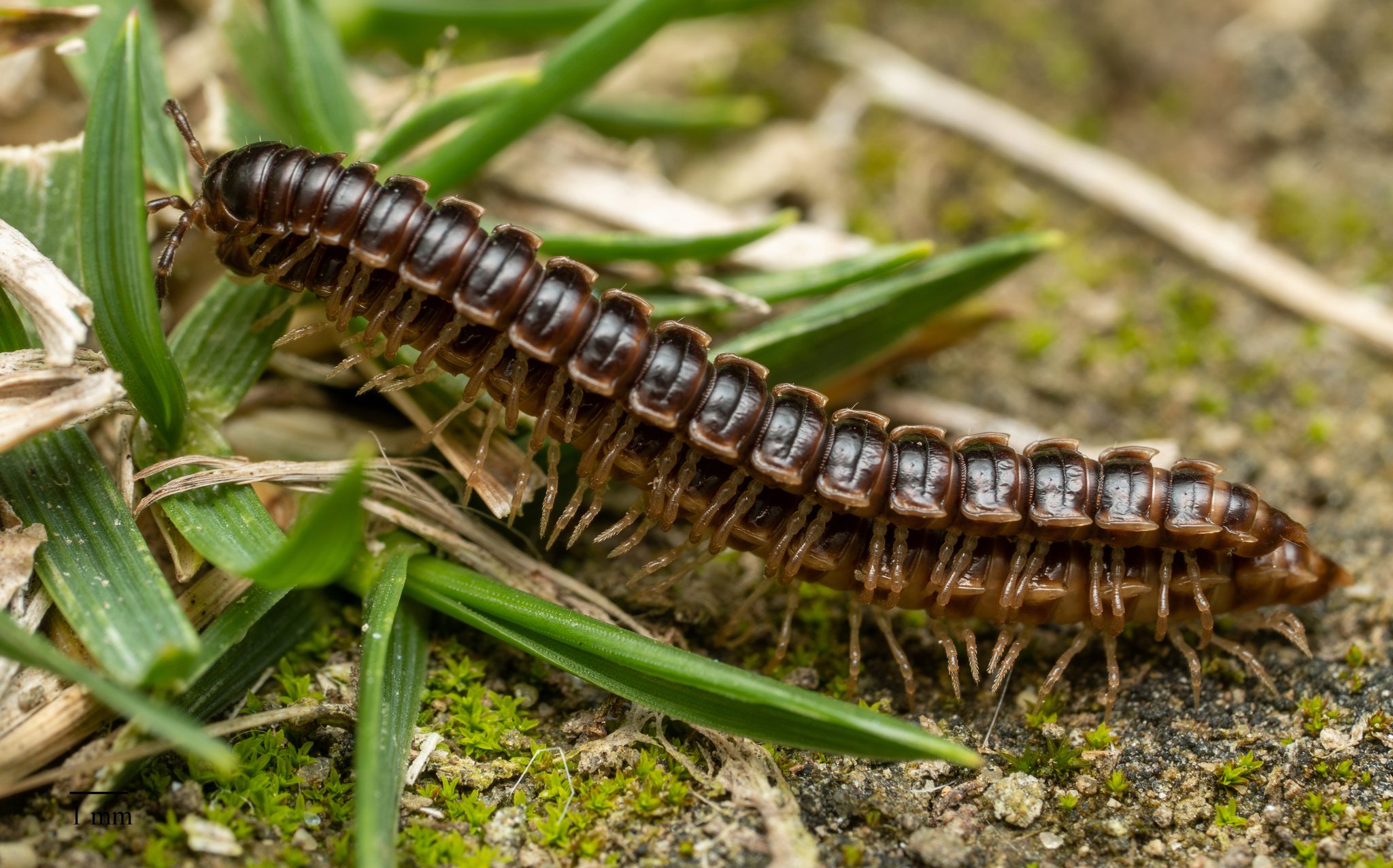This close-up photograph, taken outdoors in what appears to be a forest or garden setting during the daytime, prominently features two brown centipedes layered on top of one another. The centipedes, nestled against a surface of dirt or rock adorned with patches of bright green moss, exhibit elongated, segmented bodies covered with dark brown ridges and numerous pointy, beige or translucent legs. The centipedes are positioned with their heads on the left and bodies extending to the right, with the lighter-colored legs appearing almost see-through in some areas. Among the ground's natural textures, slim green leaves and some light brown, dead leaves provide additional earthy context, particularly visible on the left side of the image. The background of the photograph fades into a blur, emphasizing the detailed appearance of the centipedes and their immediate surroundings.